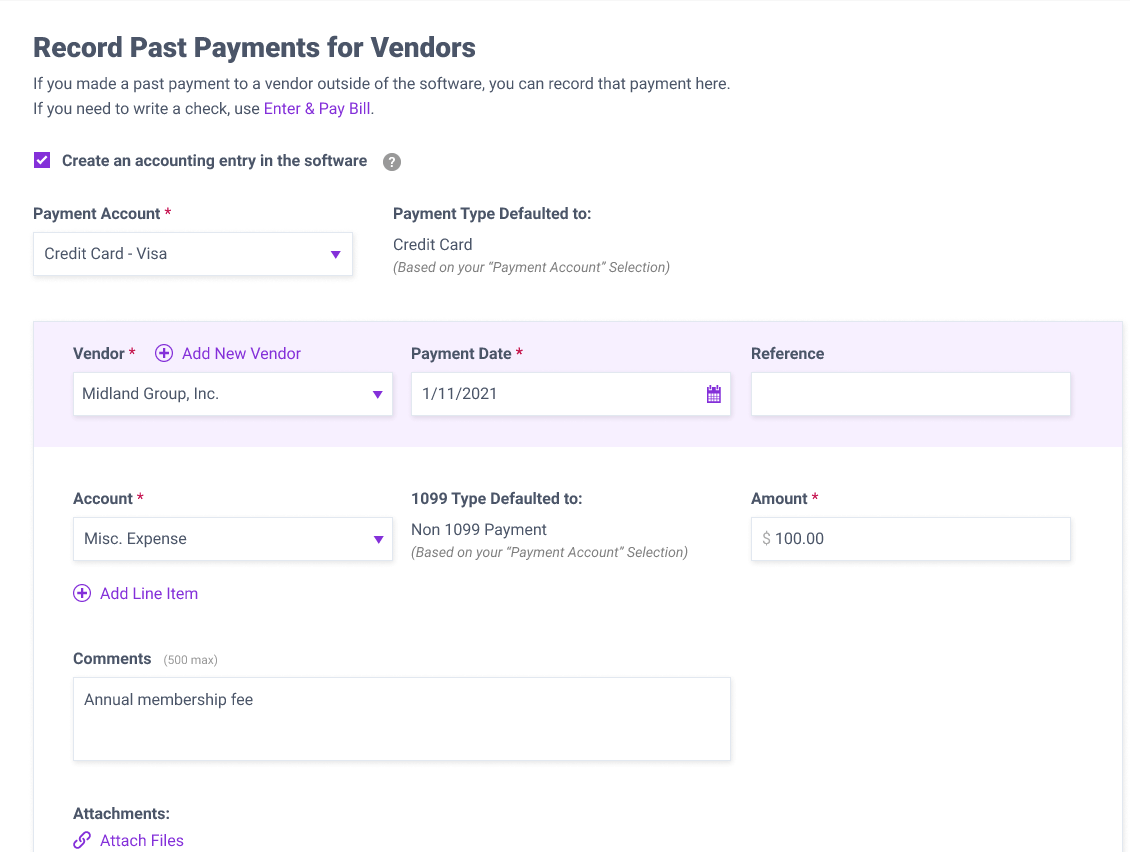**Detailed Caption:**

The webpage interface is designed for recording past vendor payments in the system. At the top of the screen, a header reads "Record Past Payments for Vendors." Below the header, there is a description that instructs users on the process: "If you made past payment to a vendor outside of the software, you can record the payment here. If you need to write a check, use Enter and Pay Bill."

Beneath the description, there is a checked checkbox labeled "Create an accounting entry in the software" with a question mark tooltip for additional information. The fields that follow are part of the payment recording form:

1. **Payment Account**: Set to "Credit Card - Visa" by default based on user selection.
2. **Payment Type**: Automatically defaulted to "Credit Card" as per the chosen payment account.
3. **Vendor**: A dropdown list with "Midland Group, Inc." selected.
4. **Payment Date**: Entered as January 11th, 2021.
5. **Reference**: An additional text box for entering reference details.
6. **Account**: Selected from a dropdown list, displaying "MIS" (likely short for Miscellaneous Expense).
7. **1099 Type**: Defaulted to "Non-1099 Payment."
8. **Amount**: Entered as $100.
9. **Comments**: Contains the note "Annual membership fees."

Lastly, the interface includes a section labeled "Attachments," which shows a logo and the word "Attached Files," indicating that users can add relevant files to the payment entry. This comprehensive layout ensures that all necessary details are captured for accurate accounting and record-keeping.